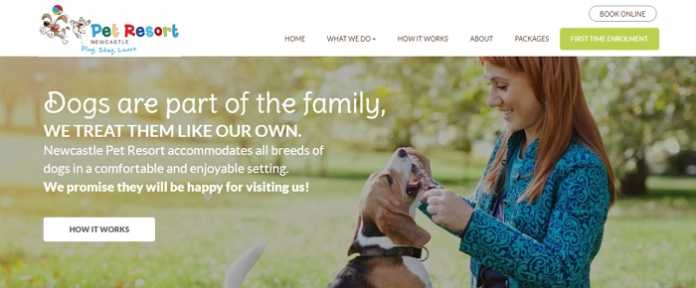Screenshot of the homepage of a website for a pet resort. The header features a white background with a vibrant cartoon illustration of two dogs with brown ears on the far left. The left dog is jumping upwards towards a multicolored ball above it. To the right of the illustration, bold, child-like text spells "PET RESORT," with each letter in alternating colors of blue, green, yellow, and red. Moving further to the right, there is negative space followed by a navigation menu with all-caps gray text displaying the options: HOME, WHAT WE DO, (with a gray downward arrow), HOW IT WORKS, ABOUT, and PACKAGES. Next to the menu, there's a lime-green box with unreadable white text due to blurring. Further right, a white pill-shaped button with a thin gray outline contains the words "BOOK ONLINE" in all-caps gray text.

Beneath the header, a vibrant photograph stretches across the page. It captures a woman in a brightly patterned blue shirt with long red hair, holding both hands towards a sitting dog in a grassy field. Background elements include green trees and a noticeable sunburst lens flare from the top left. Overlaid on the image is white text that reads, "DOGS ARE PART OF THE FAMILY." Below in all-caps, "WE TREAT THEM LIKE OUR OWN." Further down, smaller white text in three lines states, "NEWCASTLE PET RESORT ACCOMMODATES ALL BREEDS OF DOGS IN A COMFORTABLE AND ENJOYABLE SETTING." Another bold line of white text follows, declaring, "WE PROMISE THEY WILL BE HAPPY FOR VISITING US." At the bottom, a white box contains dark gray text that reads, "HOW IT WORKS."